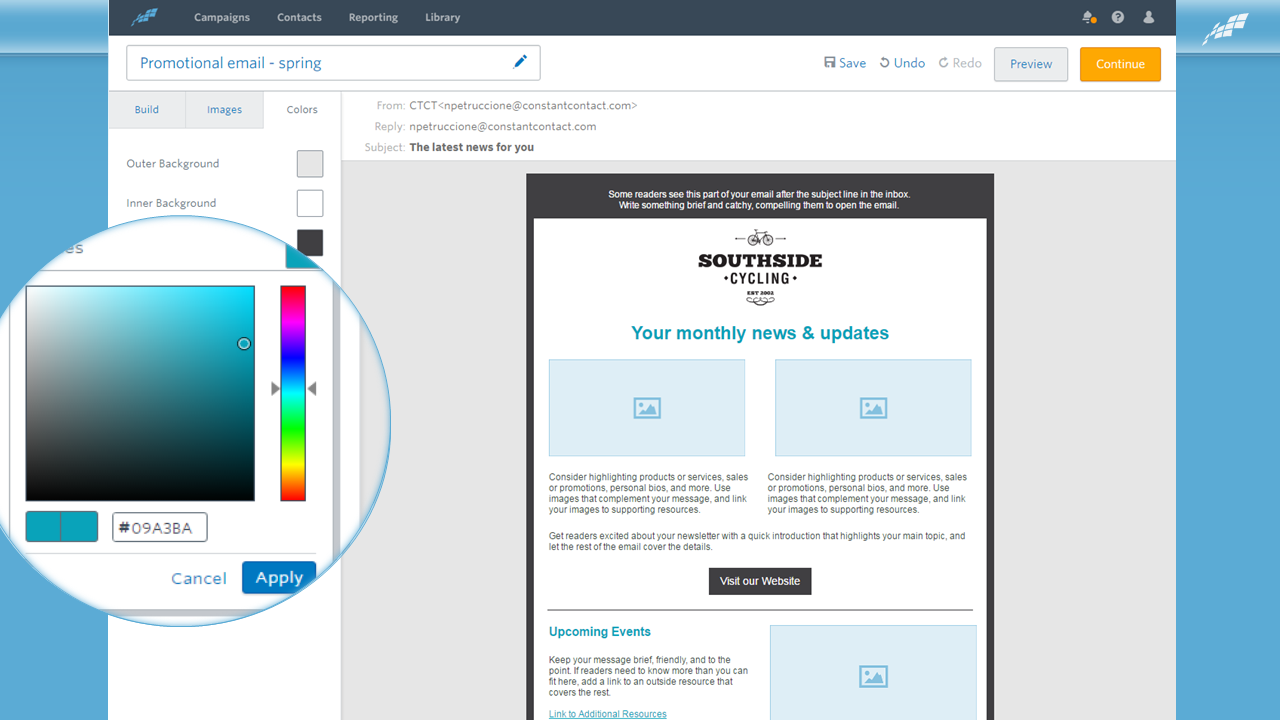A marketing professional is deep in their creative process, crafting a promotional email newsletter for the spring season. The focus is on a centered mock-up displayed on what appears to be Microsoft Word or Open Office. The email's header reads "South Side Cycling: Your Monthly News and Updates," accompanied by a small bicycle silhouette, hinting at its target audience of cycling enthusiasts. To the left of the mock-up, a robust color wheel interface is open, with adjustments being made to a blue-gray palette. The RGB color value being fine-tuned is 09A3BA. The workspace features several open windows, indicating a Windows operating system environment. On the screen, additional sections such as "Order," "Build," and "Images" are visible, contributing to the email's content and design. The attention to color and detail is crucial as the professional ensures the newsletter's aesthetic aligns perfectly with the spring theme and brand identity.